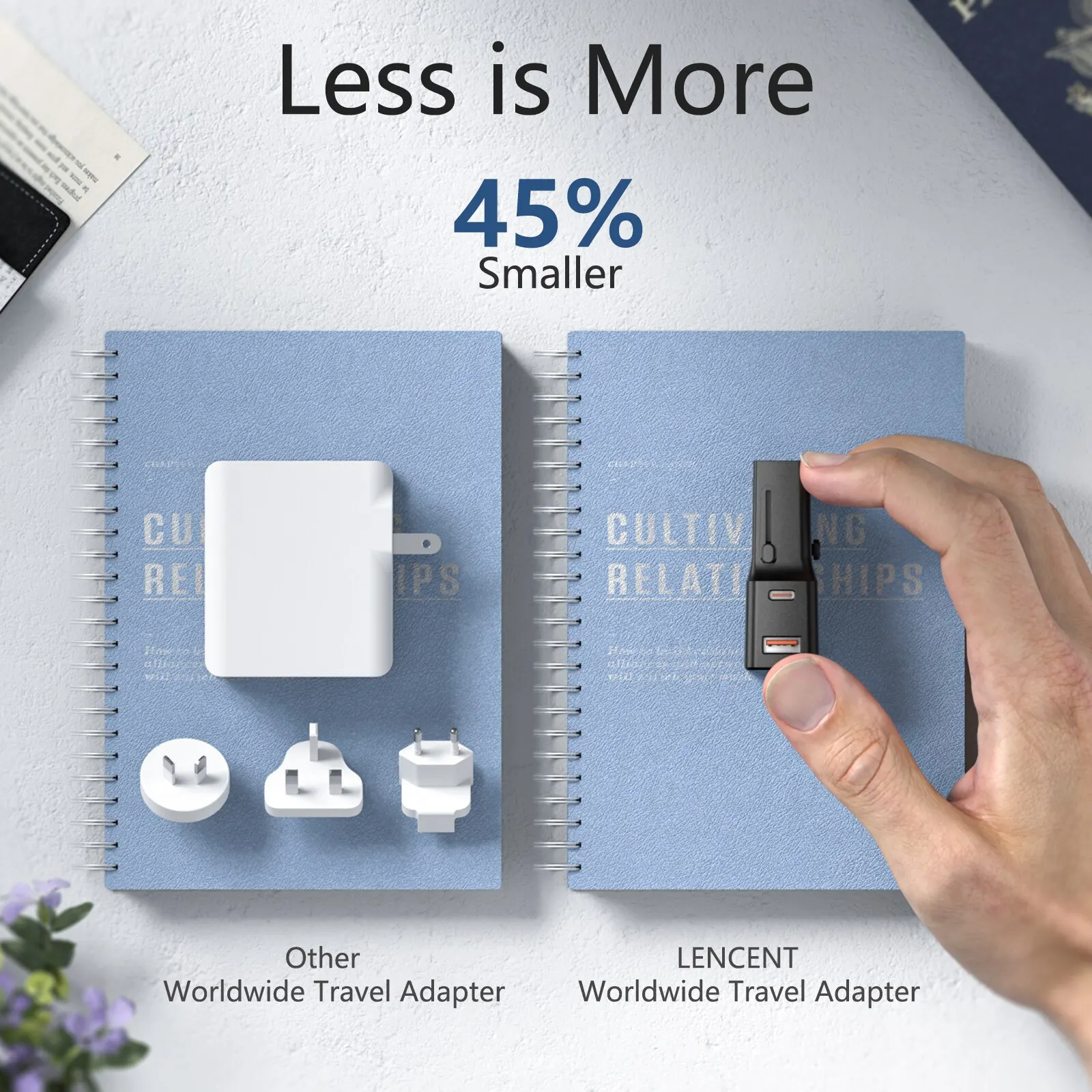The advertisement image showcases a gray background with the prominent text at the top, "Less is More" in black letters, followed by "45% Smaller" in blue and black letters. The focal point is two light blue, spiral-bound notebooks with silver coils positioned side by side. The cover of the notebooks includes the text “cultivating relationships” in light silver font. The left notebook features a white rectangular adapter with three different plugs beneath it, denoted as "Other Worldwide Travel Adapter." On the right, a Caucasian hand holds a sleek, black, narrow rectangular adapter labeled "LensScent Worldwide Travel Adapter." Both notebooks rest on a white surface. The advertisement emphasizes the compact and efficient design of the LensScent adapter, suggesting it is 45% smaller and more convenient for travel compared to traditional adapters.